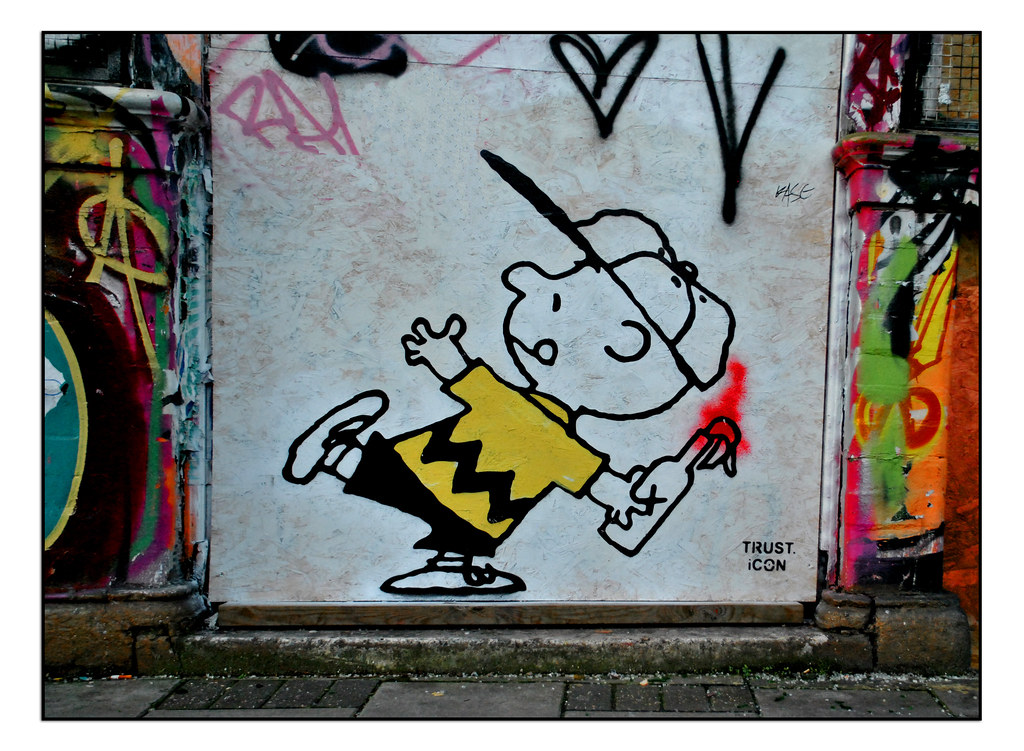The image depicts vibrant outdoor graffiti on a grimy urban wall, heavily adorned with a medley of colors—green, yellow, pink, red, orange, and blue. The focal point, however, is a striking depiction of Charlie Brown situated in the center of the wall, where the background is mostly painted white. Charlie Brown is illustrated with his trademark yellow shirt featuring a black zigzag pattern, black shorts, and white shoes. His character is captured mid-action, leaning back on one foot, with his tongue out in concentration, and poised to throw a Molotov cocktail. The bottle in his hand is clear, marked with an X, and has a rag stuffed in the top, which is ablaze. Charlie Brown is also adorned with a baseball cap, white with a black trim. Surrounding this central piece, the wall is covered with various graffiti, including multi-colored splashes and squiggly pink letters. A prominent black heart is visible above Charlie Brown, and in the bottom right corner, the words "Trust Icon" are inscribed in black lettering. The urban setting is emphasized with details of a dirty street littered with cigarette butts, adding to the gritty ambiance.